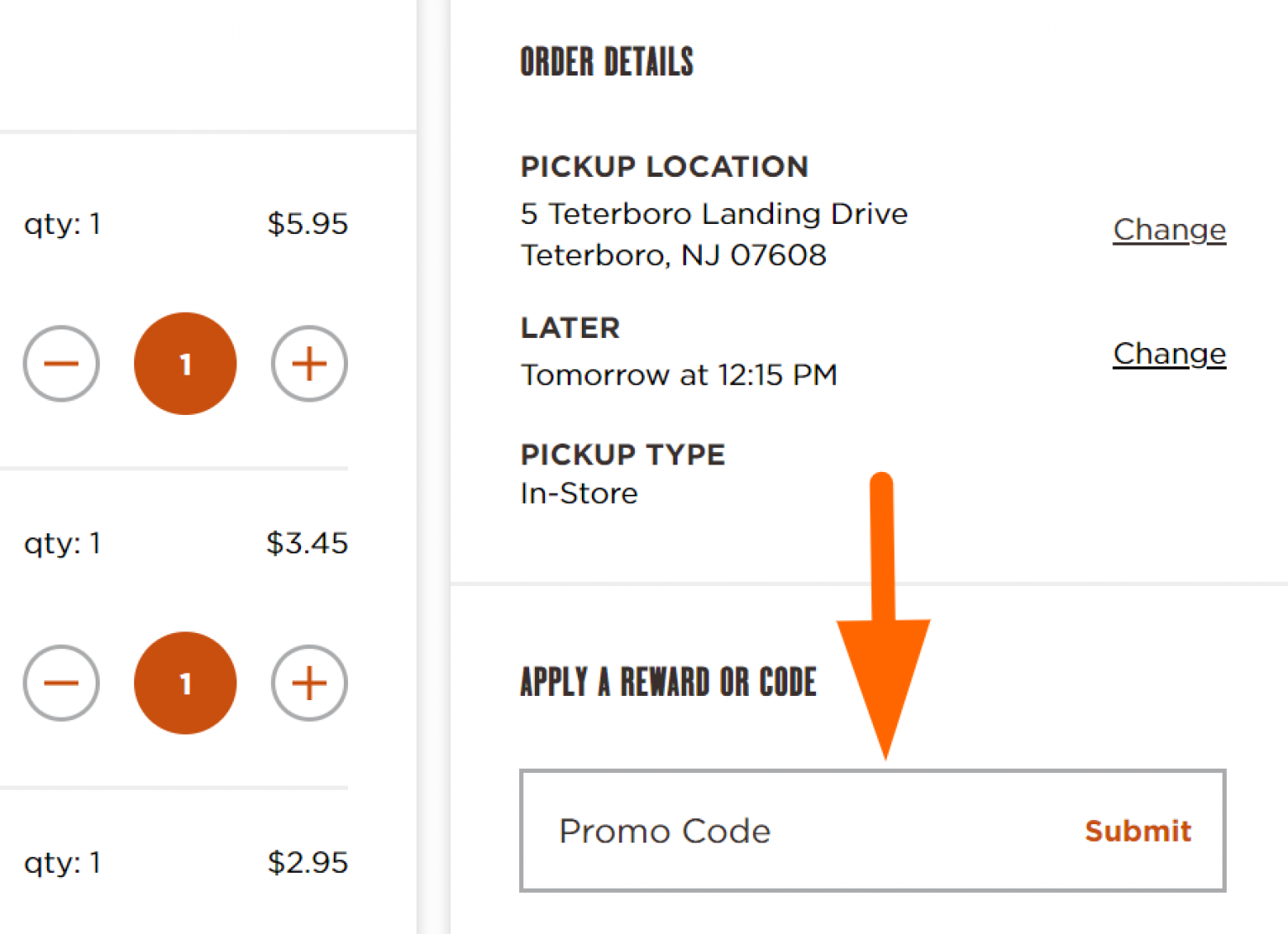The image is divided into two sections, with the section on the left being narrower than the section on the right. 

In the narrower left section, at the top, it displays "Quantity: 1" and "595" on the right. Between these details, there is an orange circle with the number "1" inside it. To the left of this circle, there is a grey circle with a minus symbol (-), and to the right, a grey circle with a plus symbol (+).

Below this, there is another entry showing "Quantity: 1" and "345" on the right. Similarly, an orange circle in the middle also houses the number "1," flanked by a grey circle with a minus symbol (-) on the left and a grey circle with a plus symbol (+) on the right.

Further down, there is the text "QTY 1, $2.95." On the right side of the broader section, it reads "Your pickup location, order details: 5 Teterboro Landing Drive," followed by "Later tomorrow at 12:15 PM." Beneath this, the text indicates the "Pickup type: In-store."

Below all this, there's a call to action, "Apply a reward or code," accompanied by an orange arrow pointing straight down. Adjacent to this is a box labeled "Promo Code," ending with a "Submit" button on the right.